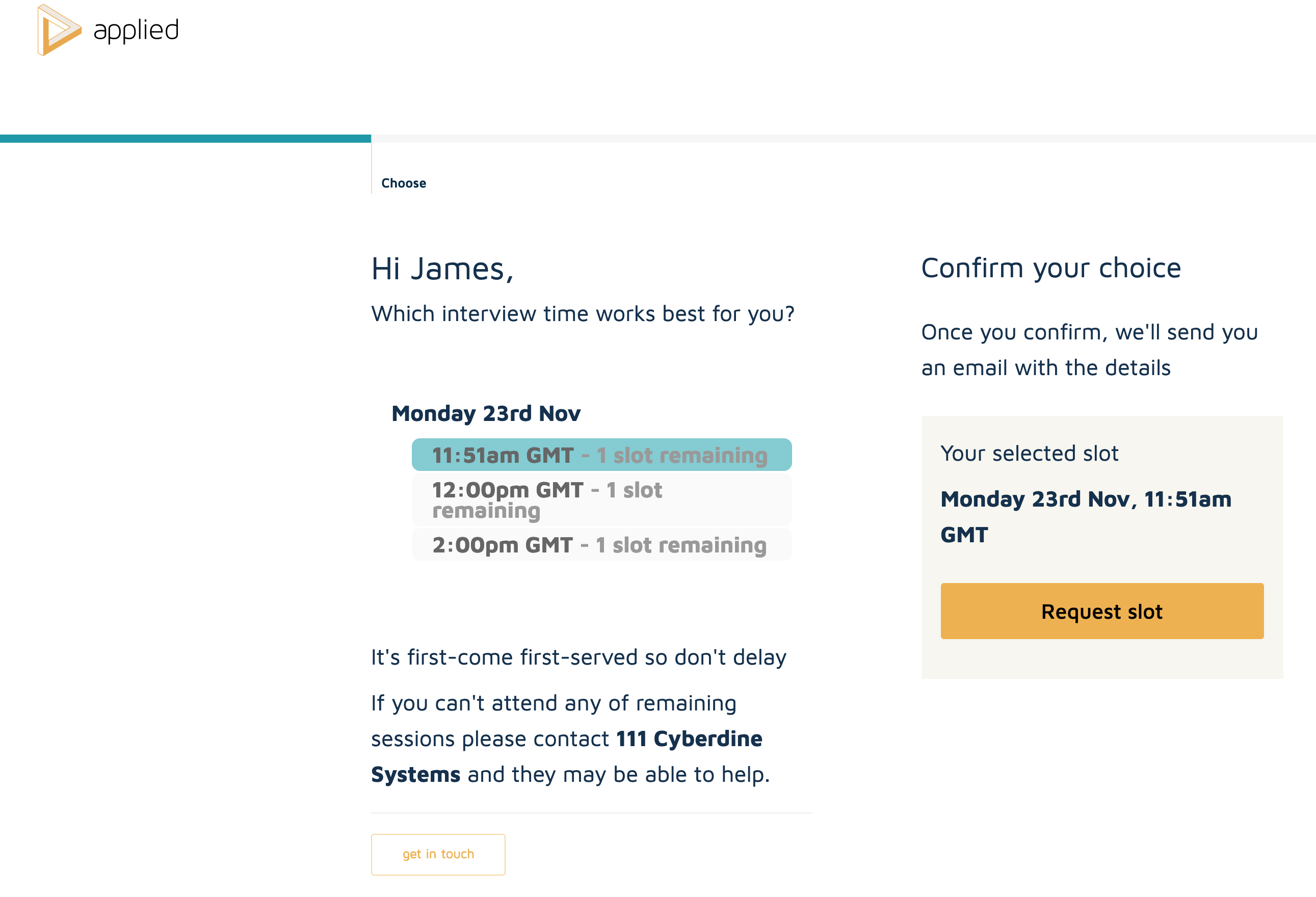This image showcases the interface of an application called "Applied." The app’s title, "Applied," is prominently displayed on the left side of the screen accompanied by a blue line, indicating a selected section, while a gray line on the right signifies an unselected section. Below the title, the interface is divided into two main sections.

The first section greets the user with "Hi James." The second section prompts the user to confirm their interview time choice, stating, "Which interview time works best for you?" Beneath this prompt, there are three available time slots for the specified interview date, Monday, 23rd of November. The times listed are 11:51 AM GMT, 12:00 PM GMT, and 2:00 PM GMT, with only one slot available for each time.

The selected time is 11:51 AM GMT, as indicated outside the selection box, confirming the choice for the interview on Monday, 23rd of November at 11:51 AM GMT.